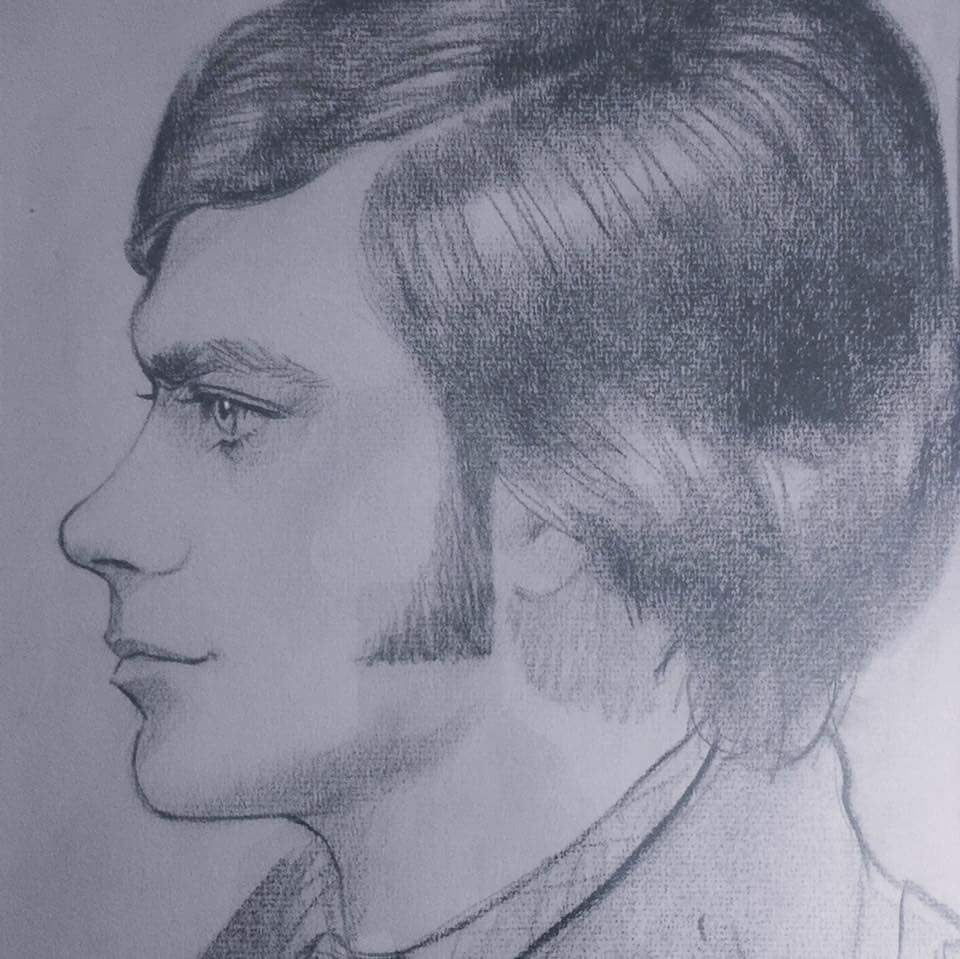This is a meticulously crafted pencil drawing on a gray piece of paper, showcasing a young male figure in a vintage style reminiscent of the 1960s or 1970s. The subject is portrayed in profile, facing to the right, allowing the viewer to observe the left side of his face in detail. His hair is parted on the left and styled to swoop gracefully over his forehead, giving off a distinctly 70s vibe. Adding to the retro aesthetic, he sports long, pronounced sideburns. The young man is dressed in a collared shirt, further enhancing the classic feel. Though the drawing is rendered entirely in pencil, the artist effectively uses highlighting and shading to bring depth to the piece. The expression on the subject's face is solemn, with a slight hint of sadness, contributing to the evocative nature of the artwork.